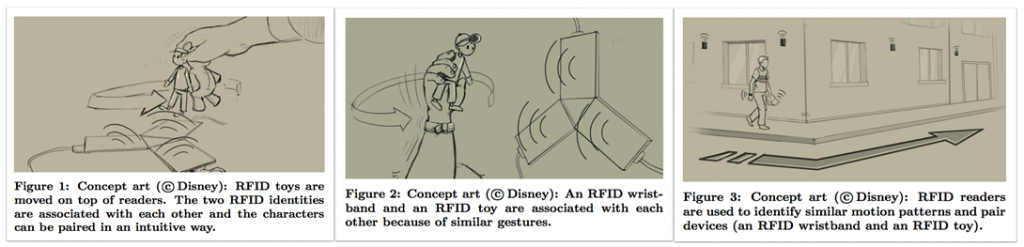This is a series of three detailed concept art panels, labeled "Figure One," "Figure Two," and "Figure Three," each with identifying text beneath them and marked as "concept art copyright Disney." The drawings are on tan paper and executed in a line sketch style. 

In the first panel, a hand is shown holding two small toys, possibly stuffed bears or dolls. The text reads, "RFID toys are moved on top of readers," indicating an interaction between the toys and RFID technology. 

The second panel depicts a hand holding a toy, described as possibly a small doll with a ball cap, which is being associated with an RFID wristband. The accompanying text explains that "an RFID wristband and an RFID toy are associated with each other due to similar gestures."

The third panel features a person walking on a sidewalk that curves around a building, indicated by an arrow. The text suggests that "RFID readers are used to identify similar motion patterns in paired devices," reinforcing the technological theme.

Each panel is accompanied by descriptions that detail the functionalities and interactions made possible by RFID technology in an intuitive and character-driven manner.